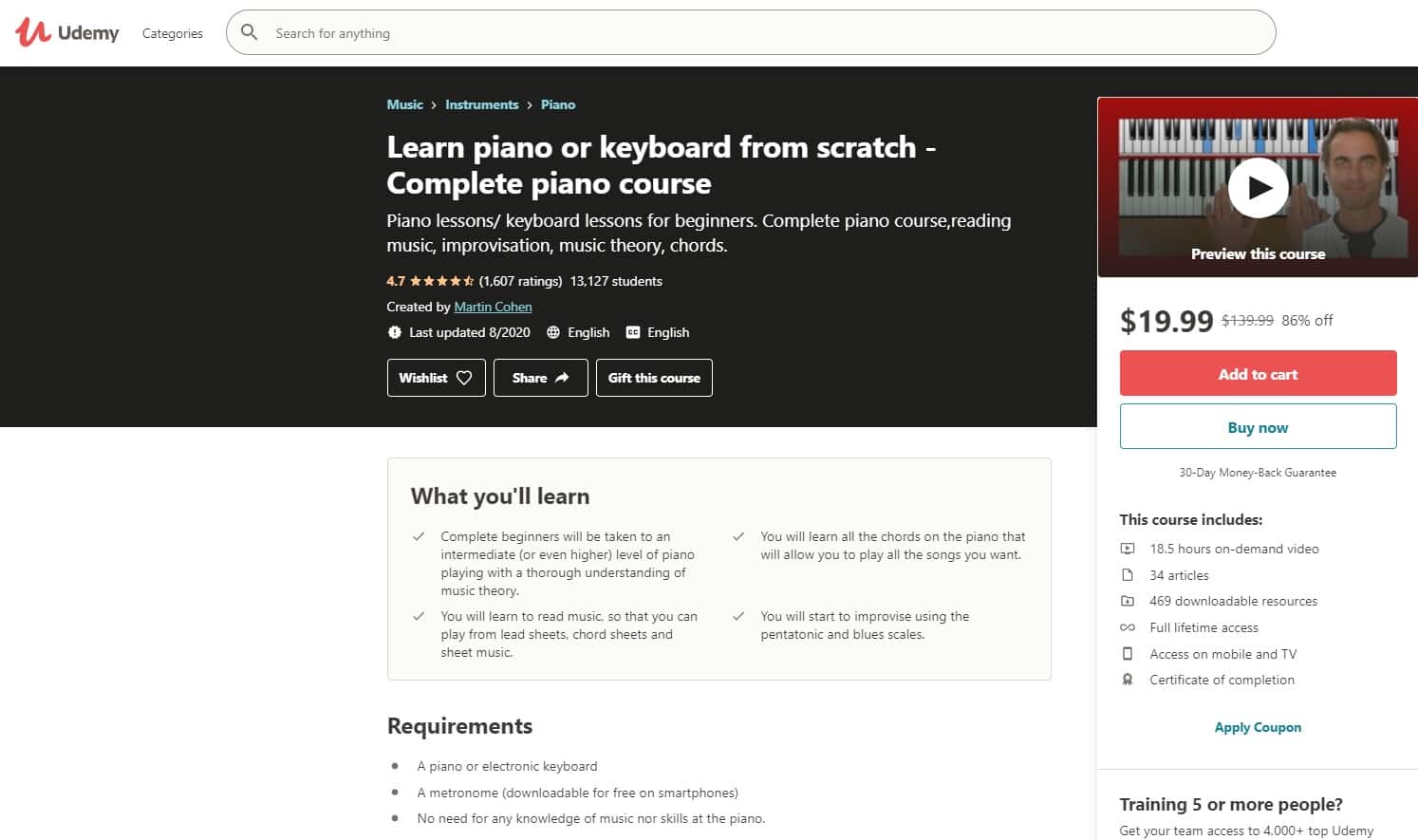This image is a landscape-mode screenshot taken likely from a laptop, featuring the Udemy website. In the upper left corner, the distinctive Udemy red logo and the word "Udemy" are clearly visible beside the "Categories" option. Centrally placed is a search bar with the prompt "Search for anything."

The main section of the image is set against a black background and prominently displays a course advertisement titled "Learn Piano or Keyboard from Scratch." It describes the offering as a "Complete Piano Course" suited for beginners, covering piano lessons, keyboard lessons, reading music, improvisation, music theory, and chords. Above the title, in blue text, are the categories: "Music, Instruments, Piano."

The course boasts an impressive rating of 4.7 gold stars from 13,000 students. Below the rating are various buttons allowing users to add the course to their wishlist, share it, or gift it. To the right, there is a video thumbnail with the option to "Preview this course."

The course is priced at $19.99 and has purchasing options– "Buy now" – paired with a 30-day money-back guarantee. It includes 18 hours of video content, 34 articles, 469 downloadable resources, lifetime access, and can be accessed on mobile and TV devices. Additionally, a certification of completion is provided upon finishing the course.

The subsequent text segment outlines the course learning outcomes, stating that complete beginners will be guided to an intermediate or higher level of piano playing, gaining a thorough understanding of music theory. Students will learn to read music, enabling them to interpret lead sheets, chord sheets, and sheet music. The course promises to teach all the essential piano chords, empowering students to play a wide variety of songs and to start improvising with pentatonic and blues scales. To enroll, learners need a piano or electronic keyboard and a metronome, with no prior knowledge required.